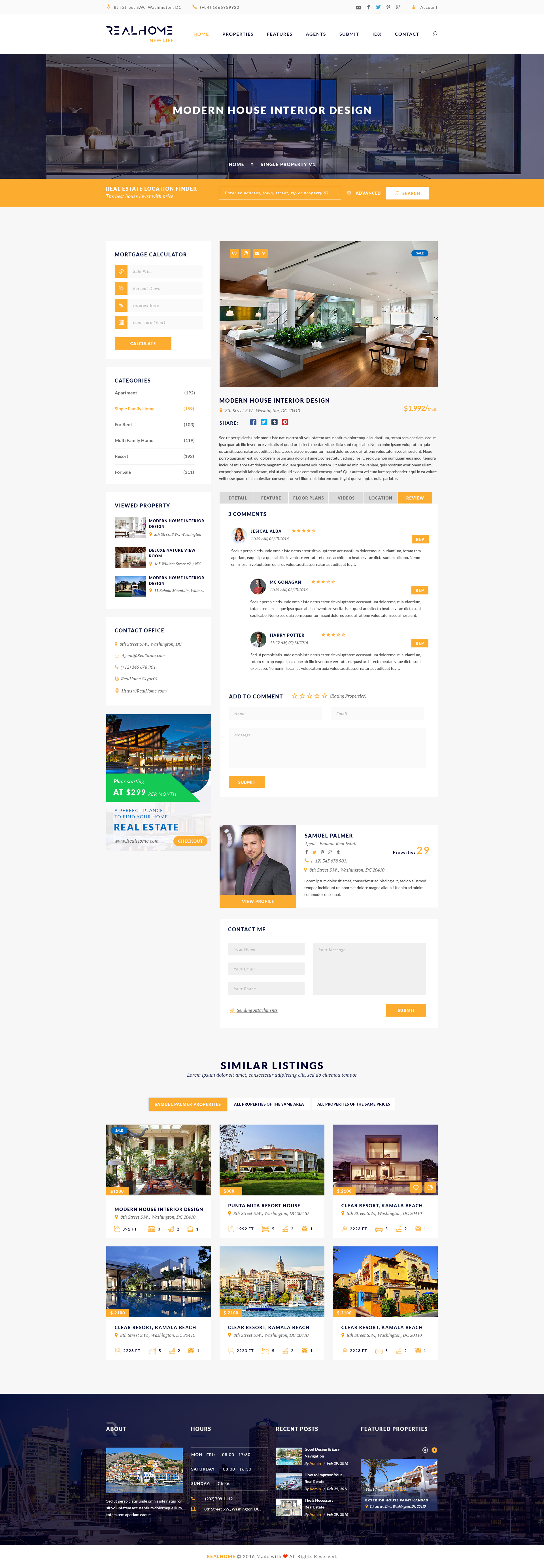A screenshot of a website shows a predominantly pale grey background. At the very top of the site, there is a white navigation bar featuring the website's name on the top left and six navigation buttons. Below this, a dark banner spans the width of the screen, with a faint image in the background and white text overlaid. Directly beneath this banner, an orange strip runs horizontally with a single white word on the right-hand side.

The main content of the website is centered, leaving large blank spaces to the left and right. On the right side of the content area, there is a photograph, accompanied by a caption and comments below. A left-hand column runs parallel to the main content. Further down the page, another article appears with a photograph and some information.

Towards the bottom of the screen, there are six thumbnails arranged in two rows of three. The website's footer is a dark navy block, containing two large thumbnails and three smaller ones, and likely includes information such as contact details, the website address, and an email address.